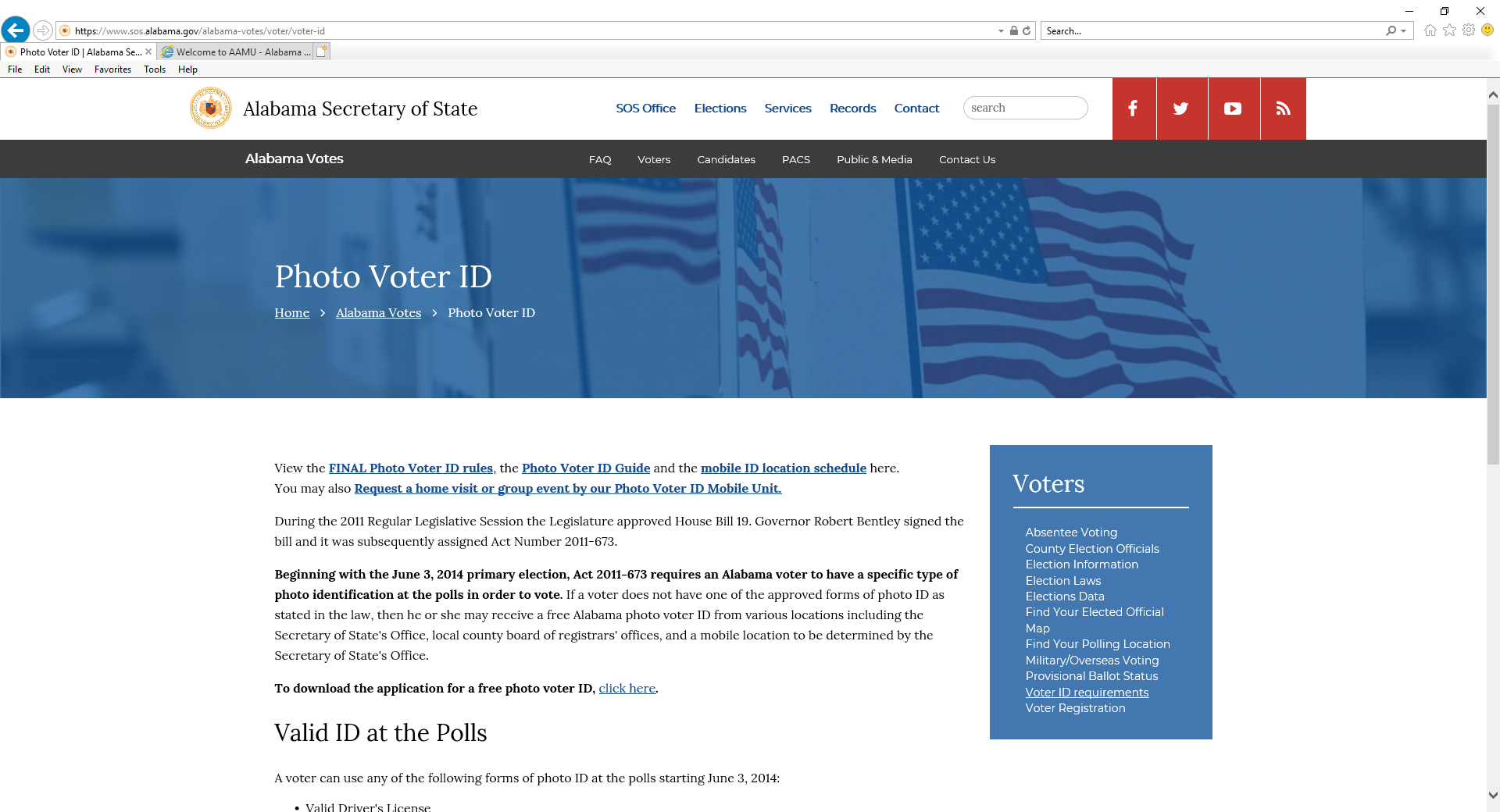A screenshot captures a desktop or laptop computer displaying a web browser window. In the top left corner, a blue circle with a white arrow pointing left is seen, followed by a white circle with a small arrow pointing right. Adjacent is a white URL box outlined in gray, next to a white search box with "search..." in black text and a gray magnifying glass icon. To the right of this search box, there is a dropdown arrow. 

Above the URL and search boxes are the browser's control buttons: minimize, maximize, and close ('X'), all rendered in black. Immediately below, a gray-outlined house icon, a star, a gear for settings, and a yellow emoji face are visible. On the far left are two browser tabs; the selected tab is white with black text, while the unselected one is gray with black text. Below the tabs, six black text menu options are listed horizontally: File, Edit, View, Favorites, Tools, and Help, separated by a thin gray horizontal line.

Prominently featured in the middle of the browser window is the text "Alabama Secretary of State" in black with a yellow seal icon beside it. There are blue text options presented in the middle, flanked by red social media rectangles with white vertical line dividers. The center showcases a large, blue, transparent background featuring the United States flag with "Photo Voter ID" written in bold white text across it.